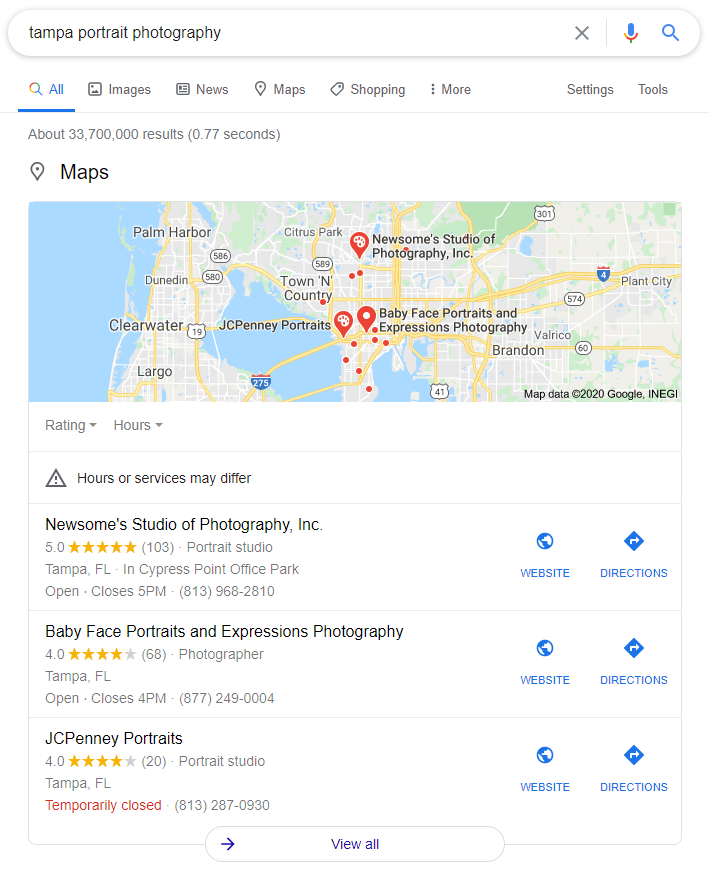A Google Maps screenshot displays search results for "Tampa portrait photography." The search bar at the top reveals "All" is selected among various tabs like "Images." The page indicates approximately 33,700,000 results found in 0.77 seconds. Beneath this is a small map highlighting several photography studios in Tampa, Florida, with red markers indicating their locations. The map is followed by three featured entries:

1. **Nuisance Studio Photography Inc.**: Rated with five gold stars.
2. **Babyface Portraits and Expressions Photography**: Rated with four stars.
3. **JCPenney Portraits**: Also rated with four stars, but noted as "Temporarily Closed" in red text.

Each entry includes links for the respective websites and directions, displayed in blue. The background is predominantly white, with text primarily in gray except for highlighted elements like the gold star ratings and the "Temporarily Closed" notice for JCPenney Portraits. At the bottom, a "View All" link is available in blue.